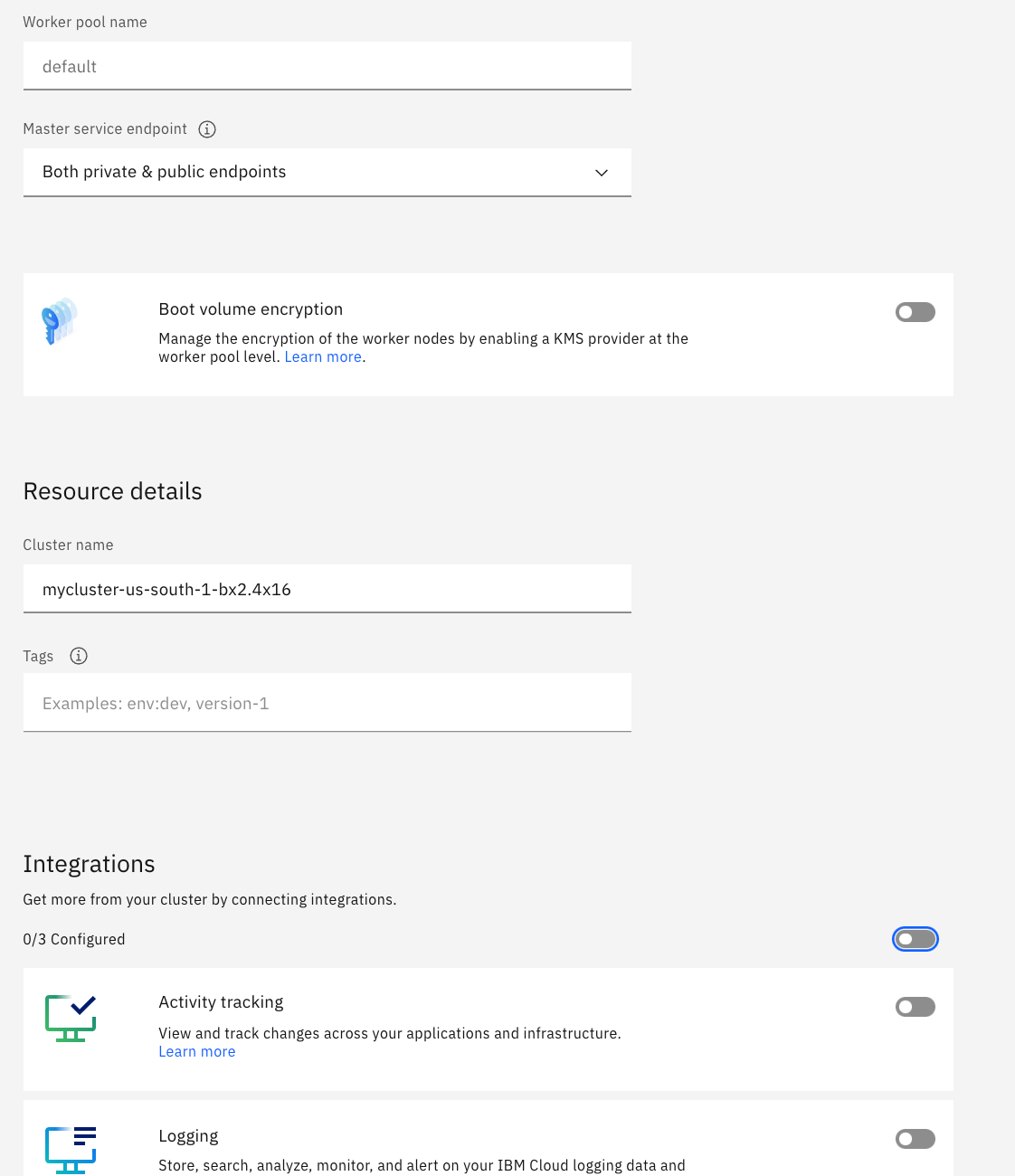**Options Menu Overview:**

The screenshot showcases an extensive options menu with several sections, each catering to specific configuration needs.

- **Top Section: Toggle Options**
  - At the very top, there are toggle options, prominently displayed for easy access and quick adjustments.

- **Worker Pool Section:**
  - A section labeled "Worker Pool Name" in small gray font.
  - Directly below this label, there is a text input bar designated for entering the master service endpoint.

- **Endpoint Configuration:**
  - Following the text input bar, there is a dropdown menu labeled "End Points."
  - This dropdown menu offers two options: "Private" and "Public" end points.

- **Encryption Settings:**
  - A significant feature in this menu is the "Boot Volume Encryption" section.
  - This section presents a white bar with a blue key icon on the left.
  - The text adjacent to the icon reads: "Boot Volume Encryption - Manage the encryption of the worker nodes by enabling a KMS provider at the Worker Pool level."
  - The encryption feature is currently toggled off, indicating it is not enabled.

- **Resource Details:**
  - The next section is titled "Resource Details."
  - Under this section, there is a field labeled "Cluster Name" followed by an input box where a cluster name has been entered.
  - Additionally, there is another input box labeled "Tags," which allows for the input of text for tagging purposes.

- **Integrations Section:**
  - The final section in the menu is "Integrations."
  - This section is also toggleable and is currently toggled off.

**Summary:**

This options menu provides a structured approach to configuring various aspects of a system, from encryption settings and endpoint management to resource details and integrations. Each section is clearly labeled and includes input fields or toggles for easy adjustments, enhancing the user’s ability to customize their setup effectively.